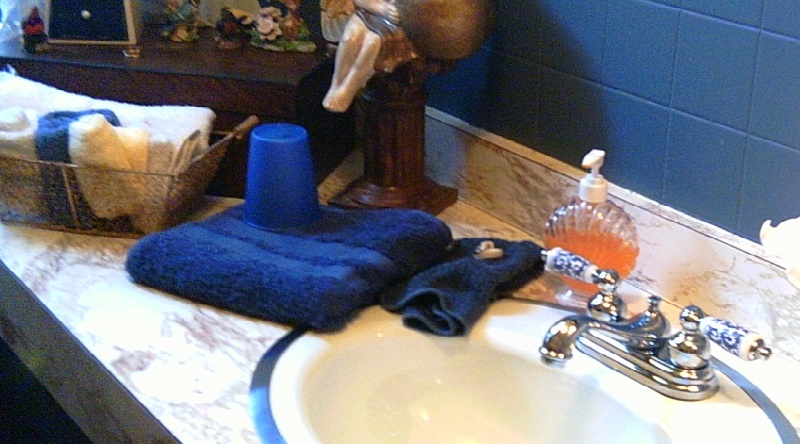This color photograph captures an elegant bathroom scene featuring a section of the sink, countertop, and wall. The upper right part of the image showcases the wall, adorned with solid blue tiles in a striking hue. In the bottom right corner, a pristine white oval sink is visible, accompanied by a sophisticated gold faucet. The faucet stands out for its exquisite white porcelain handles, which are decorated with delicate blue designs reminiscent of fine china.

Adjacent to the sink, the countertop surface appears to be crafted from luxurious marble, presenting a cream white base with intricate gray veining. Adding to the bathroom's aesthetic, a large, neatly folded royal blue towel lies on the counter, alongside a slightly darker washcloth. Atop the towel sits a blue, conical object that resembles a candle, enhancing the serene ambiance.

On the left side of the image, a brass wire basket holds an array of items, including several cosmetic bottles and a neatly folded white towel. The thoughtful arrangement and choice of elements in the photograph highlight the bathroom's sophisticated and inviting atmosphere.